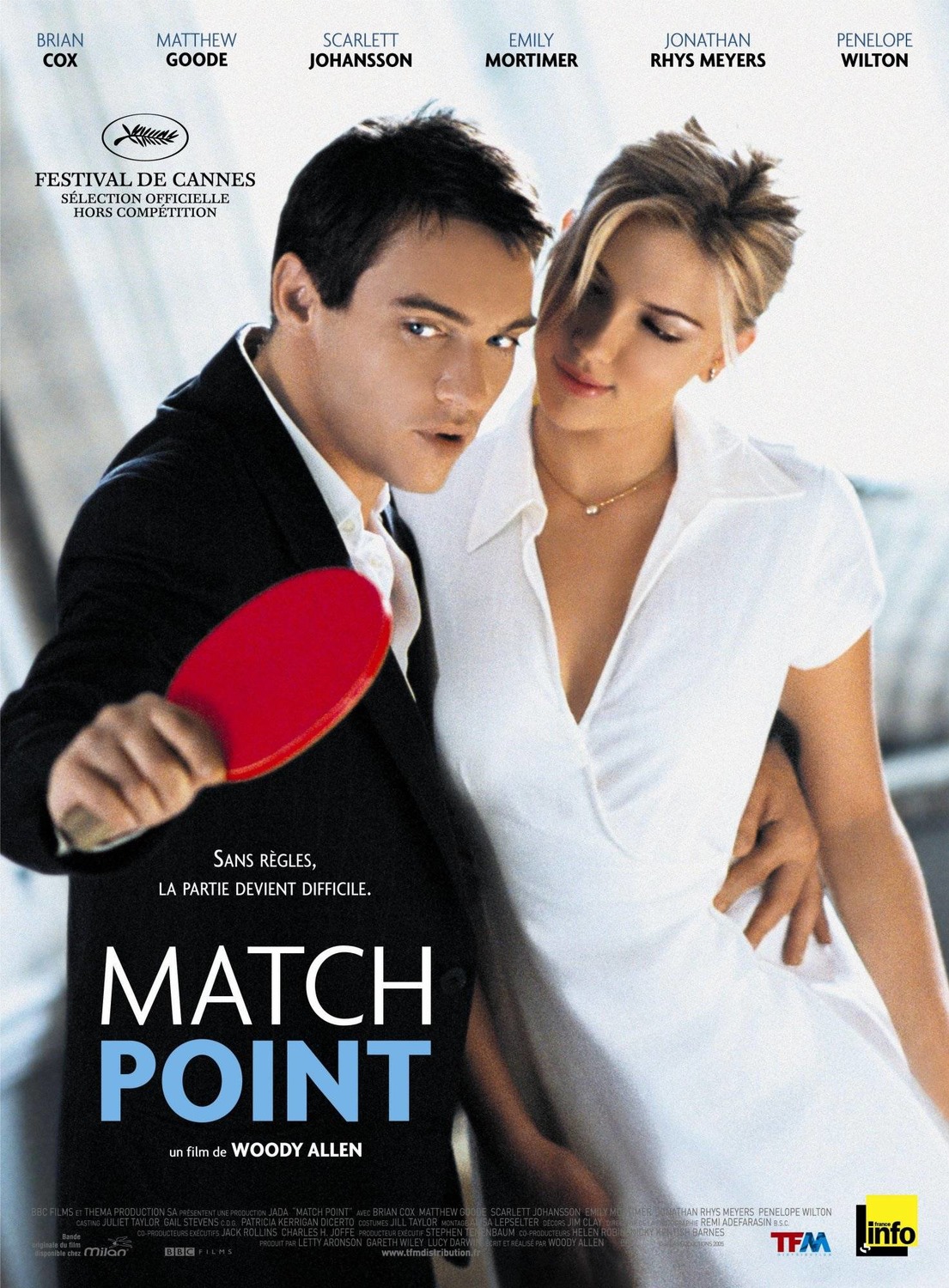This visually striking movie poster for "Match Point," directed by Woody Allen and featured at the Festival de Cannes, showcases an intimate moment between a couple. On the left, a dark-haired man is dressed in a dark blue jacket over an open white dress shirt and is holding a red ping-pong paddle in his right hand, extended towards the viewer. His left arm is wrapped around the hip of a blonde woman to his right, who is wearing a collared, open-neck white dress. Her eyes are closed, and she is looking at him, while he gazes at the paddle. The names of the cast members—Brian Cox, Matthew Goode, Scarlett Johansson, Emily Mortimer, Jonathan Rhys-Meyers, and Penelope Wilton—are listed at the top of the poster. The title "Match Point" and "Un film de Woody Allen" are displayed prominently at the lower left, with the Festival de Cannes emblem in the upper left. Both characters are cut off just below the waist in this rectangular portrait-oriented poster, creating a sense of close-knit drama and tension.